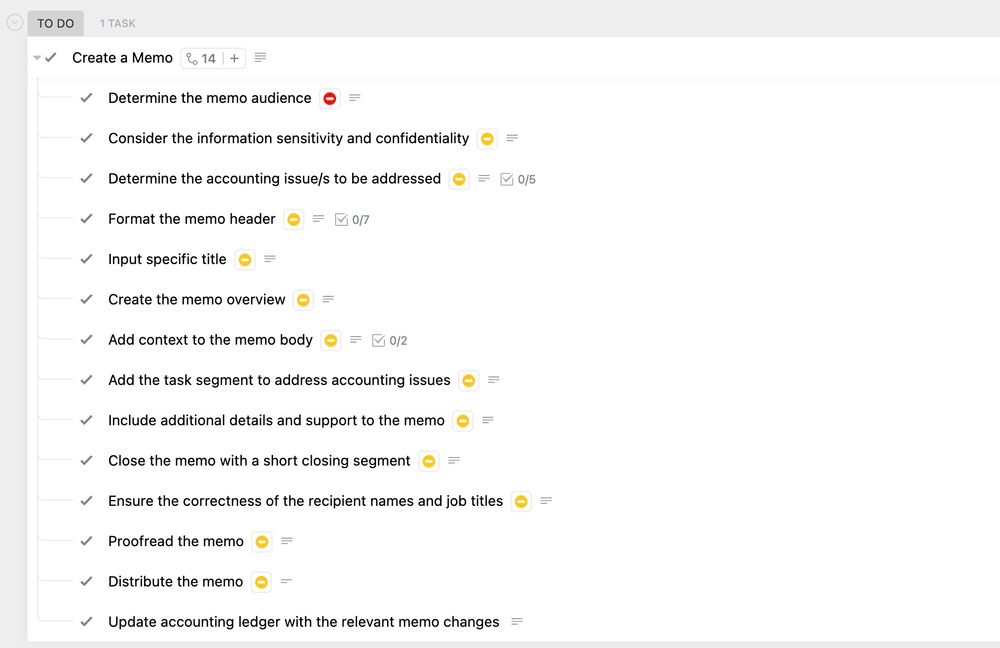This screenshot captures a computer screen displaying a detailed to-do list in a single browser tab. The tab is labeled with "To-Do List" and shows that there is "1 task" remaining. The main task, "Create a memo," is listed with a check mark to its left, indicating it has been selected. A drop-down menu reveals an extensive skills tree of sub-tasks necessary for completing the memo. 

The tasks are:
1. **Determine the memo audience** - Marked with a red circle with a line through it, indicating it has a critical status.
2. **Consider the information sensitivity and confidentiality** - Marked with a yellow circle with a line through it.
3. **Determine the accounting issues to be addressed** - Marked with a yellow circle with a line through it.
4. **Format the memo header input specific title** - Marked with a yellow circle with a line through it.
5. **Create the memo overview** - Marked with a yellow circle with a line through it.
6. **Add context to the memo body** - Marked with a yellow circle with a line through it.
7. **Add the task segment to address accounting issues** - Marked with a yellow circle with a line through it.
8. **Include additional details and support to the memo** - Marked with a yellow circle with a line through it.
9. **Close the memo with a short closing segment** - Marked with a yellow circle with a line through it.
10. **Ensure the correctness of the recipient names and job titles** - Marked with a yellow circle with a line through it.
11. **Proofread the memo** - Marked with a yellow circle with a line through it.
12. **Distribute the memo** - Marked with a yellow circle with a line through it.
13. **Update accounting ledger with the relevant memo changes** - Marked with a yellow circle with a line through it.

Each sub-task is accompanied by a check mark on the left and a square with a circle inside it on the right, emphasizing their completion status. The only sub-task highlighted in red, "Determine the memo audience," implies its special attention requirement, while the others in yellow indicate lesser but notable importance.